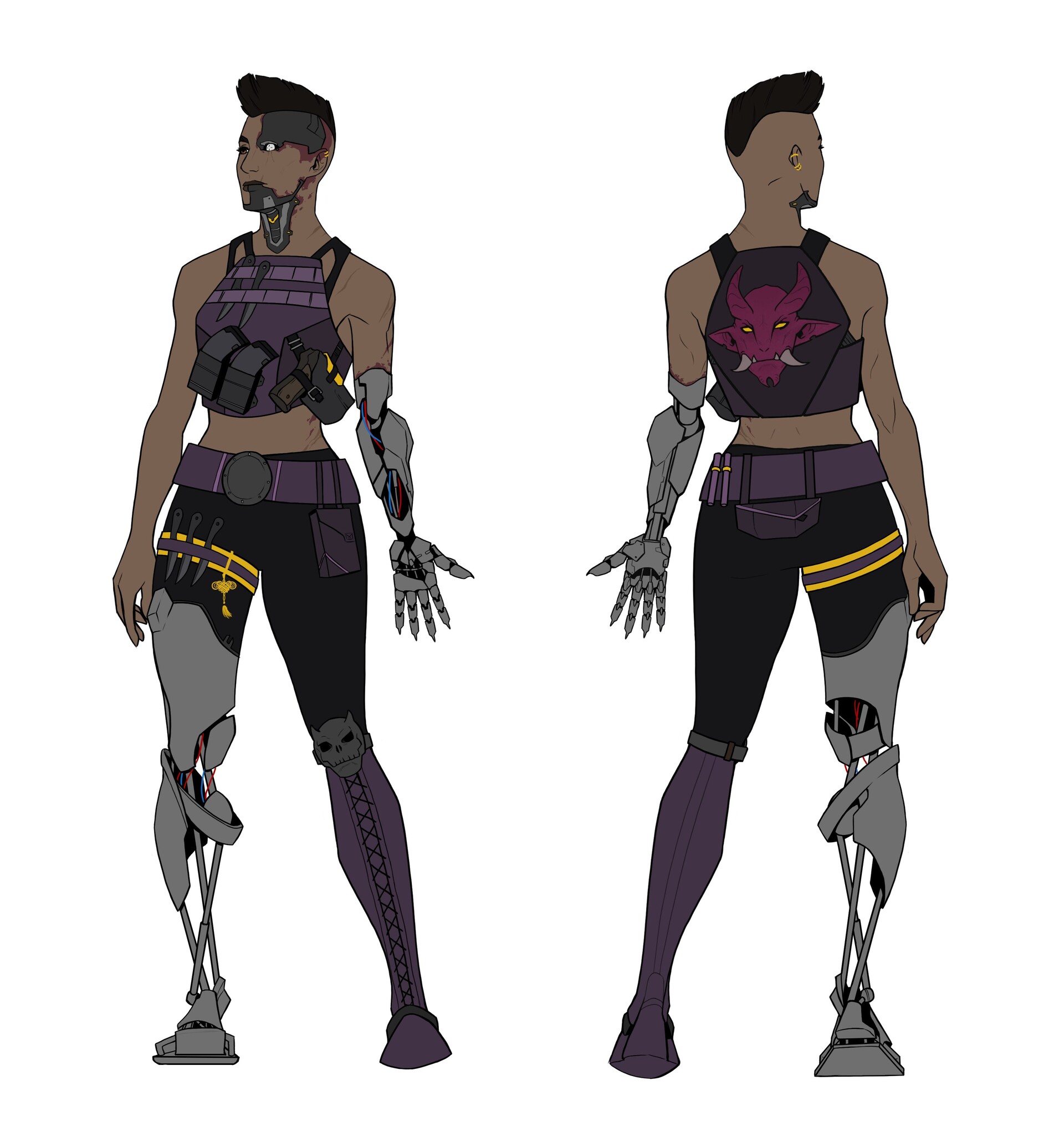This concept art is a detailed illustration of a science fiction character, potentially for a movie or video game, drawn in a comic book cell-shaded style. The central figure is an African American woman with a mohawk hairstyle. Her left eye is a bright white, contrasting with her brown right eye. She features a metal plate above her left eye and another extending from her chin down her neck, indicating cybernetic enhancements. Her right arm appears human, while her left arm is mechanical, ending in a claw and adorned with visible wires. She wears a purple top that exposes her midriff, which is equipped with ammo cartridges and a pistol. Her left leg shows a skull at the knee and ends in a purple-laced boot, whereas her right leg is entirely robotic. She is also outfitted with a wide purple belt and black pants. The art includes two views of the character: a front view and a back view. The back view reveals a red-faced demon with horns printed on her shirt, reinforcing the character's edgy, futuristic aesthetic.